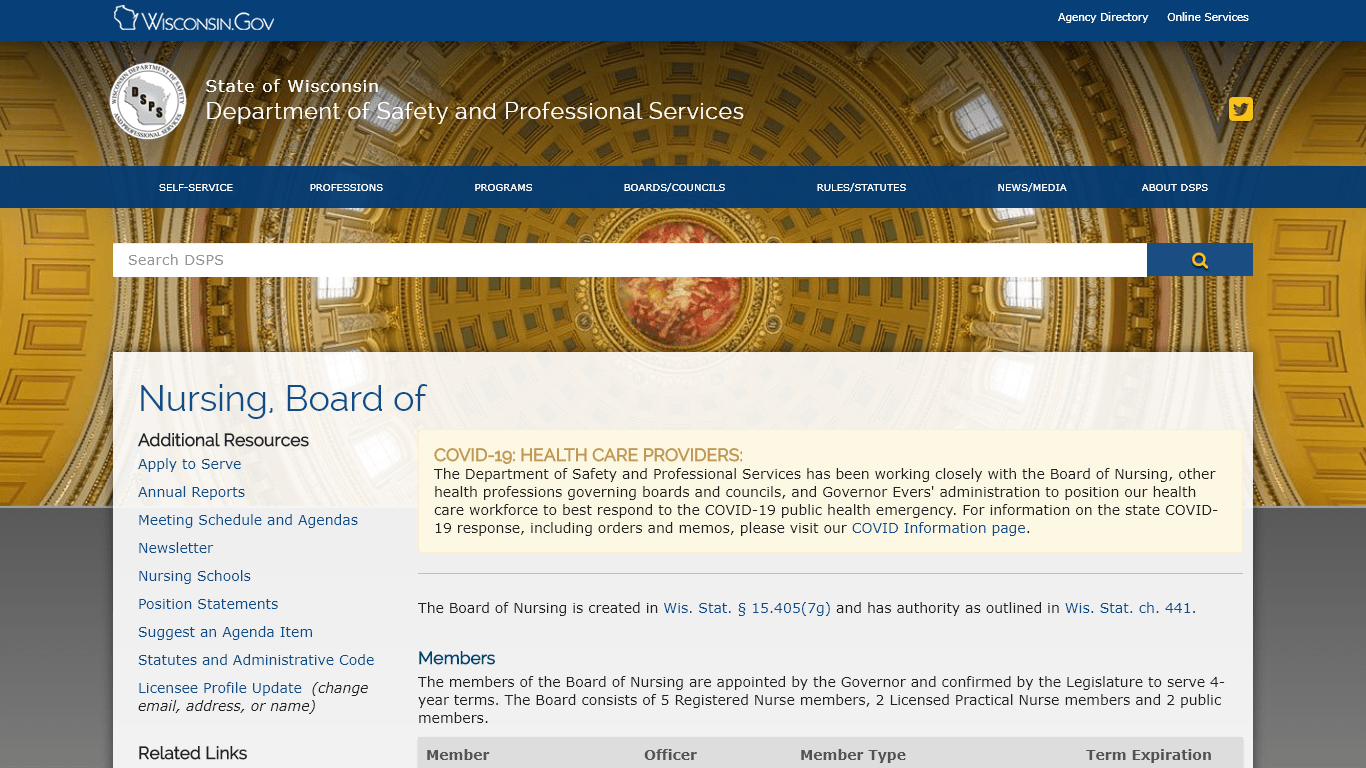The image displays a webpage header with a long blue rectangular bar at the top, featuring "Wisconsin Gov" in white text, followed by "State of Wisconsin Department of Safety and Professional Services." Below this, another blue rectangular bar contains several menu options, though they appear blurry and difficult to read. The discernible options include "Newsletter" towards the right, "About" in the center, "Board Councils" to the left of the center, "Programs" further left, and "Self Service" at the very left.

Further down is a long white search bar. To the left of this bar, within a small square, is the label "Nursing Board." On the right side, there is a section labeled "COVID-19 Health Care Providers," which offers relevant information within a rectangular box.

The text underneath mentions that the Board of Nursing is established under Wisconsin State law, specifically Chapter 441, which grants its authority. Additional options are listed on the left, including "Apply to Serve," "Annual Reports," "Newsletter," "Position Statements," "Suggest an Agenda Item," "Statuses," "Administration Code," and "License Profile Update."